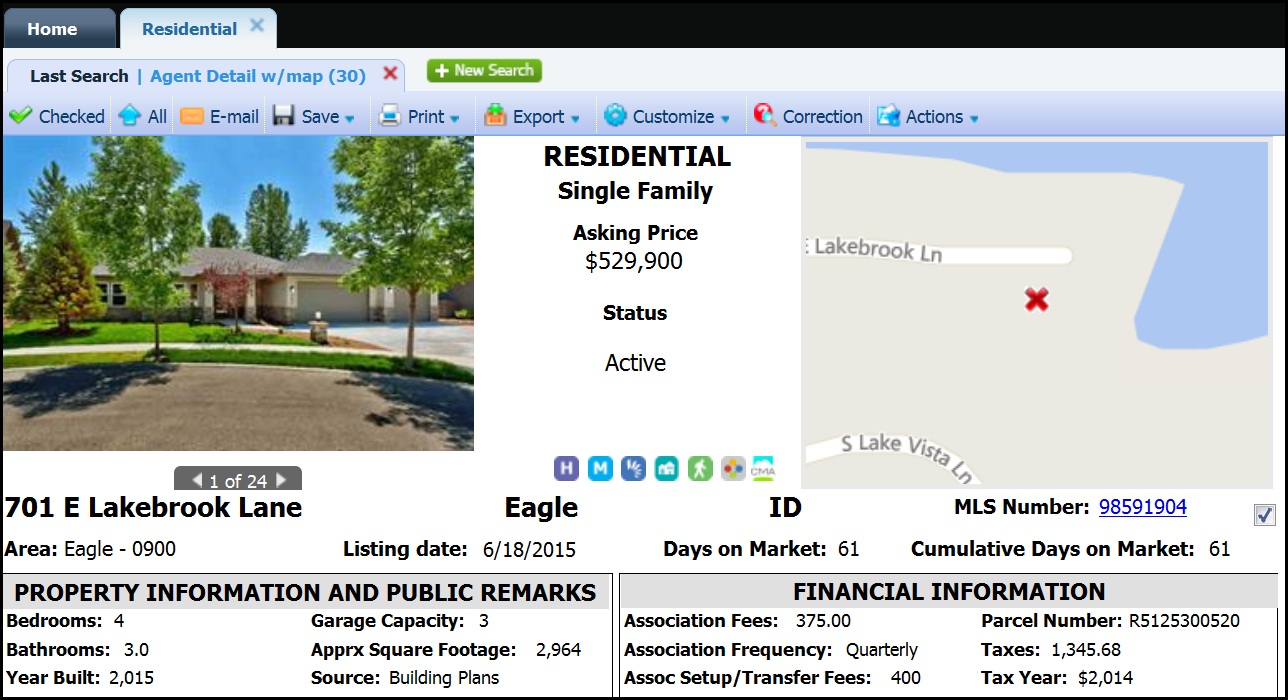In this detailed computer screenshot, the viewer is presented with a horizontal, left-to-right oriented interface, characteristic of a real estate listing platform. Across the top of the screen, a black bar houses multiple tabs, including “Home” and “Residential.” Just below this, the navigation displays the selected options: “Last Search” highlighted in black and “Agent Detail with Map (30)” in blue, with the number indicating a possible sorting parameter. 

Next to these options, there is an X icon, likely intended to close the window, accompanied by a green button for initiating a new search. Below the navigation bar, an assortment of clickable buttons with corresponding icons are present: “Checked,” “All,” “Email,” “Save,” “Print,” “Export,” “Customize,” “Correction,” and “Actions.”

At the center of the interface, the main content features a photograph of a house, marked as the first in a series of 24 images that users can scroll through. Essential property details are displayed prominently: the address, area, listing date, days on the market, MLS number, cumulative days on the market, and type — indicating it is a residential single-family home. The asking price is noted as $529,900 and its status is denoted as "Active."

A map showing the property's location is also included, providing spatial context. At the page's lower section, two elongated rectangular boxes segregate "Property Information" and "Public Remarks." These sections detail specifics such as the number of bedrooms and bathrooms, year built, garage capacity, and square footage. Financial data encompasses association fees, their frequency, setup and transfer fees, parcel number, taxes, and the relevant tax year. This comprehensive layout ensures users have access to all pertinent information at a glance.